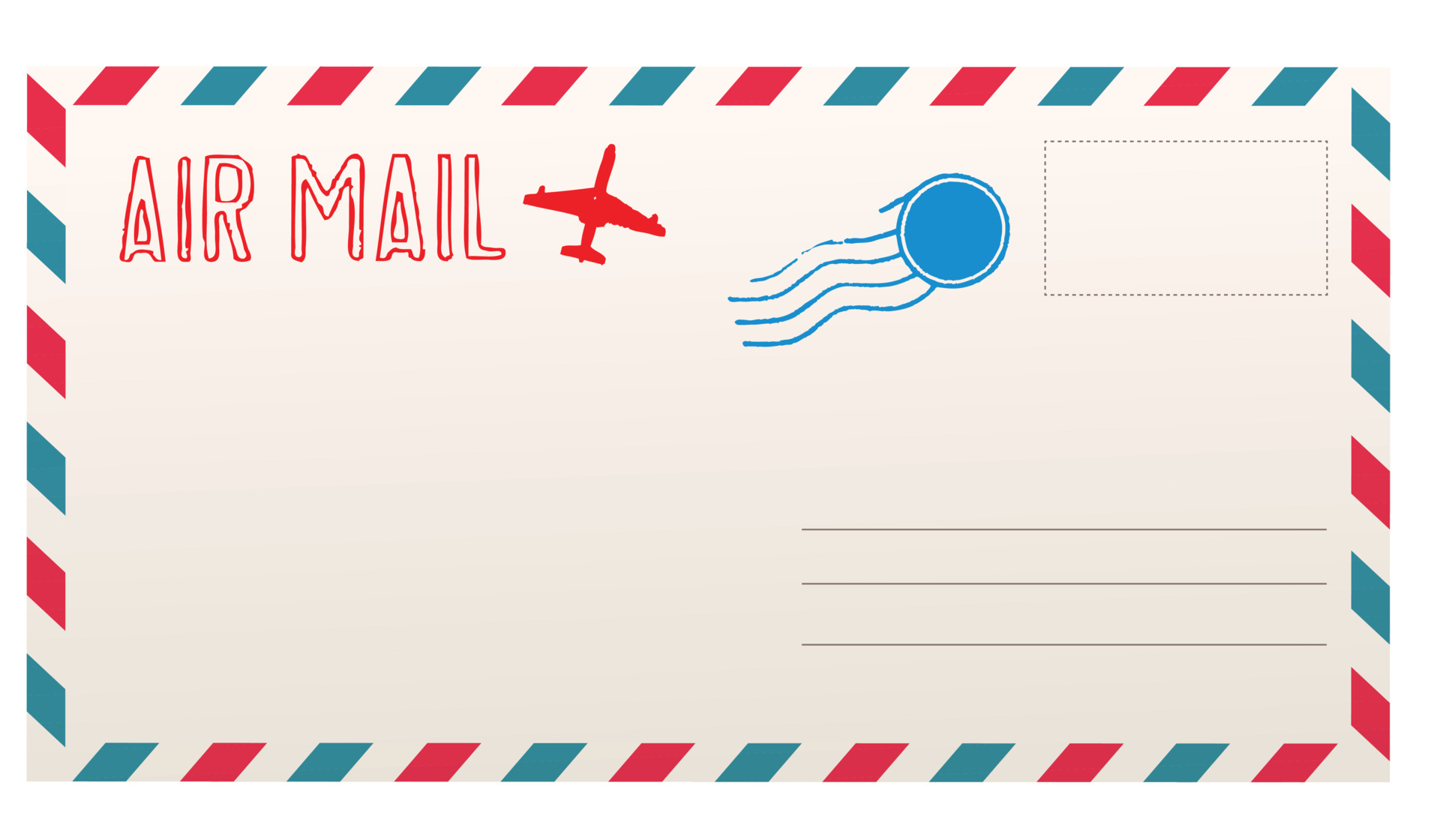This photograph features an airmail envelope with distinctive red, white, and blue diagonal stripes adorning each side, creating a vibrant border. In the top left corner, "AIR MAIL" is prominently displayed in hollow, capital letters with a red outline. Adjacent to this text, a red airplane icon, depicted from a vantage point that shows both wings, points upward. Just to the right of the airplane, a blue emblem with swirling wave patterns is visible. Further to the right is a dashed rectangle, marking the space designated for postage stamps. In the bottom right corner of the envelope, there are three horizontal lines intended for the recipient's address. The envelope’s off-white background contrasts sharply with the colorful border, making the airmail design unmistakable.